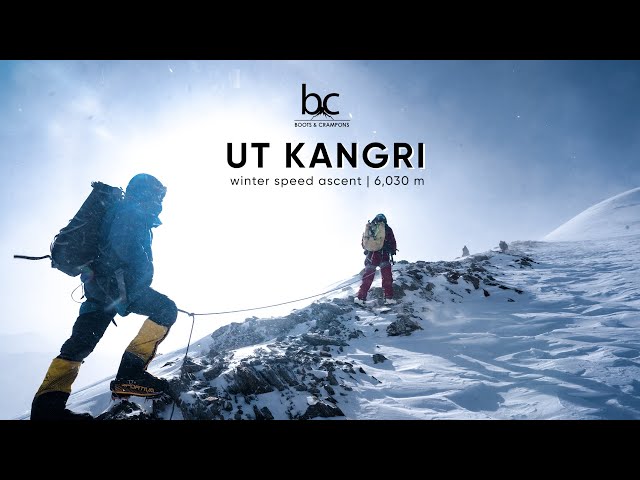This photograph captures a dramatic mountain climbing scene in a snowy, high-altitude setting. Two mountaineers, dressed in full winter gear, are ascending a rocky ridge that diagonally spans from the bottom left to the top right of the frame. The climber on the left is distinguished by a dark blue jacket, dark pants, yellow gaiters, a large dark backpack, and a hood. The second climber, positioned slightly ahead in the middle of the frame, is in red attire with a tan backpack and white boots. They are connected by a safety rope, illustrating their teamwork and cautious ascent.

The backdrop features a stark blue sky adorned with wispy white clouds, centering a blown-out sun that adds a luminous glow slightly left of center. The landscape around the climbers includes snow-covered sections, emphasizing the harsh, icy environment they are navigating. In the distance, two more climbers appear as faint gray dots further up the ridge, hinting at the scale and expanse of the mountain.

Overlaying the sky, black text reads "BC," accompanied by a mountain icon, followed by "Utkangri" in larger letters. Below that, smaller text states "Winter Speed Ascent, 6030 meters," contextualizing the scene as a high-stakes, swift mountain climb.